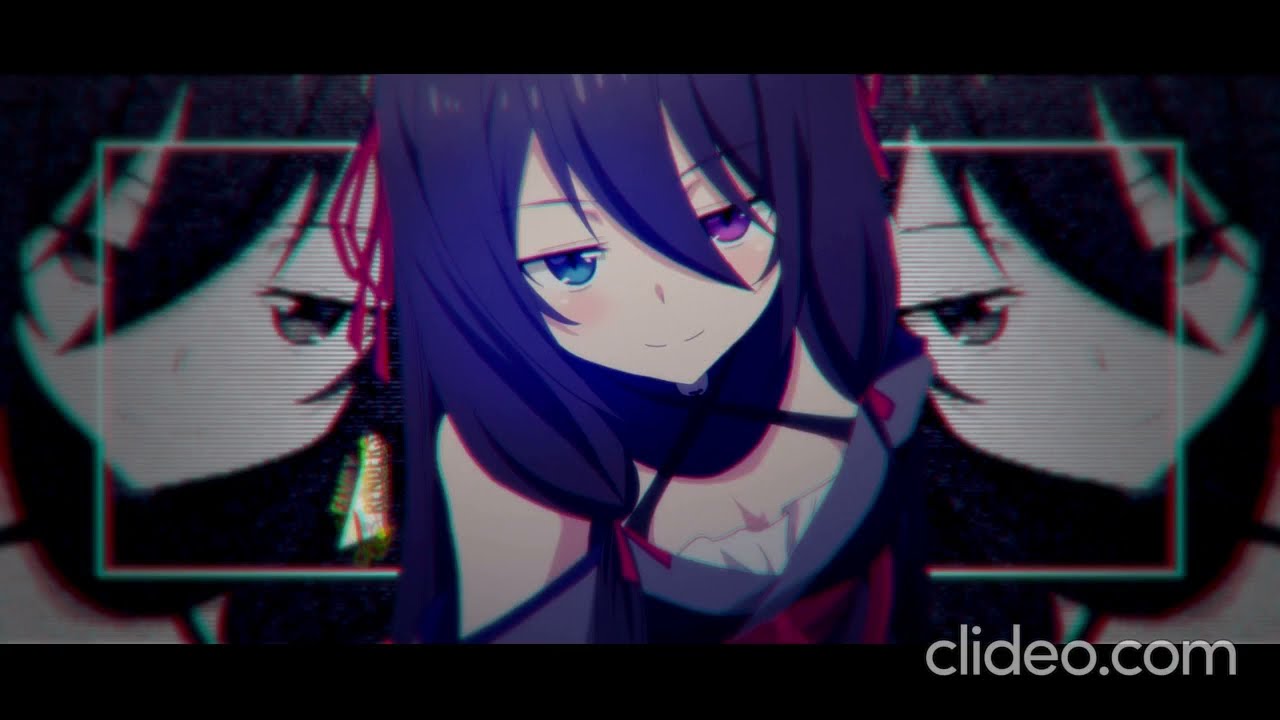In this digitally created anime-style artwork from Clideo.com, we see a central female character with long, swooping purple hair that falls in front of her face. She notably has heterochromatic eyes—one blue and one purple. She is adorned in a purple top with cross-threaded straps and white ruffle fabric covering part of her cleavage. Positioned on a black background, the image includes mirrored black-and-white versions of the character's face on the left and right sides, creating a striking visual effect. There is also a white rectangular digital focus box across the central figure and the mirrored faces, enhancing the modern, graphic design aesthetic. The only text present is "CLIDEO.com," prominently located in the bottom right corner. The colors featured prominently within the artwork are black, purple, pink, light green, and blue.